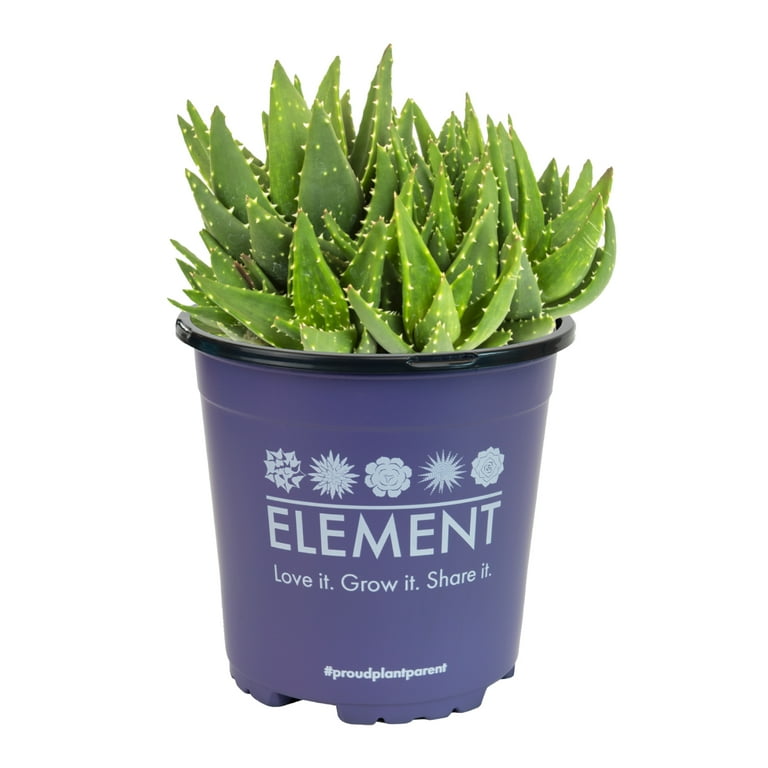The image showcases a vibrant green succulent plant, characterized by long, triangular leaves studded with small spikes. This plant is housed in a purple plastic pot, which prominently features various white cartoon flower graphics above the brand name "Element". Below the brand name is the slogan, "love it, grow it, share it." At the base of the planter, the text reads "#proudplantparent." The background of the photograph has a clean, solid color, either black or white, likely edited to eliminate distractions and emphasize the subject.